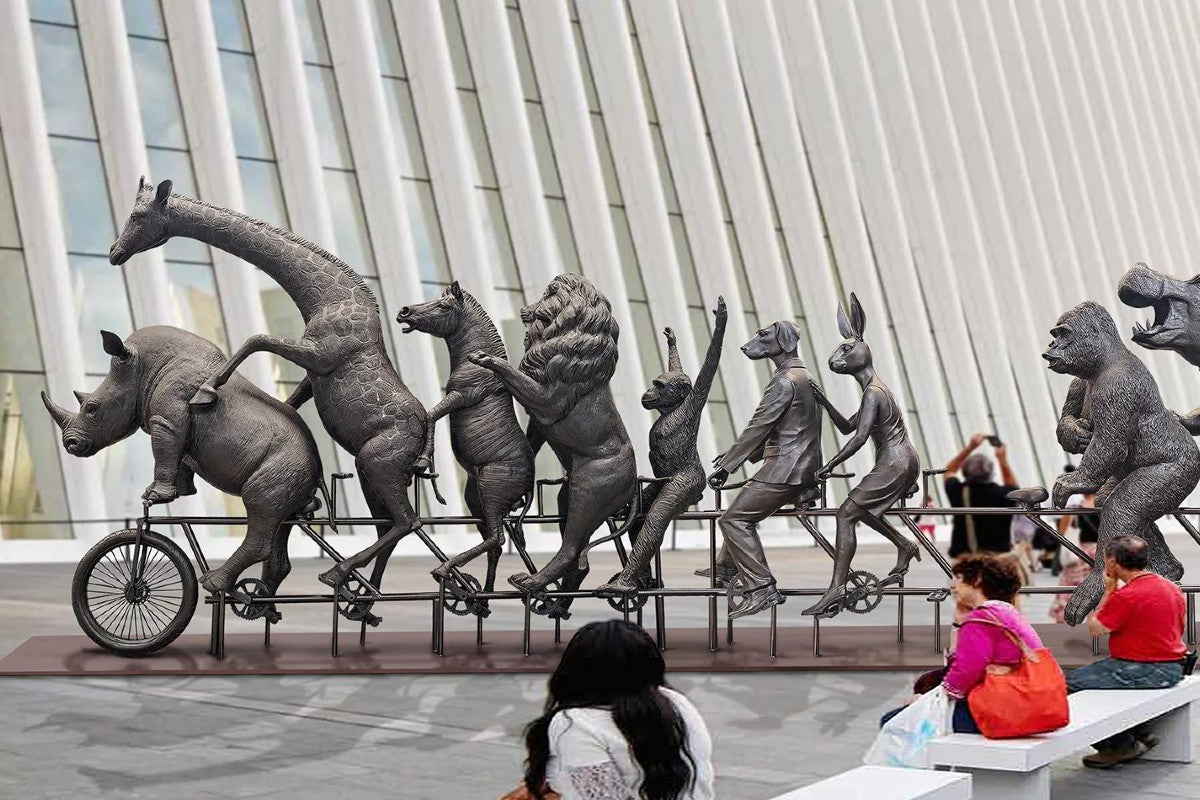In front of an architecturally intriguing, tall skyscraper with numerous windows, a bronze or metal sculpture of a multi-passenger bicycle takes center stage. The close-up photograph reveals a whimsical parade of nine different animals riding the tandem bike from front to rear: a rhinoceros, a giraffe, a zebra, a lion, a chimpanzee with its hands up, a dog in a suit, a rabbit in a dress, an ape, and a partially visible hippo. The animals appear to be connected, with most placing their hands on each other's shoulders. In the foreground, three individuals are seated on white benches, all facing the sculpture. The first is a woman with long black hair, the second a woman with short brown hair wearing a pink shirt and carrying an orange purse, and the third a man in a red T-shirt and blue pants. In the distant background, another man wearing a black shirt is seen taking a photograph of the building. The sculpture and foreground action are set against a mostly monochromatic backdrop, contrasting with the bright attire of the people on the benches, adding a burst of color to the scene.